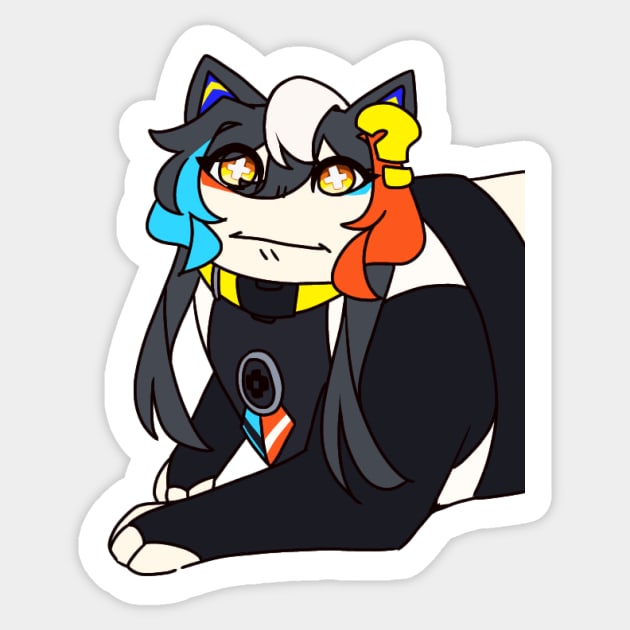This is a sticker of an anime-style cat, surrounded by a white border. The cat is primarily black with distinct features: white paws, a white stripe on the top of its head, and a white mouth area. It has vibrant hair colors, with red on the right side and blue on the left, and its ears match this scheme with one being gray and the other tipped in blue and orange. Above the right ear, there's a yellow question mark. The cat has large, round eyes that are yellow with white crosses in the center. It wears a yellow collar with a black clasp and a medal on its chest decorated with red and blue ribbons. The cat is laying down, with one paw fully on the ground and the other slightly raised, as if leaning partially on it. The sticker is set against a grayish-white background.